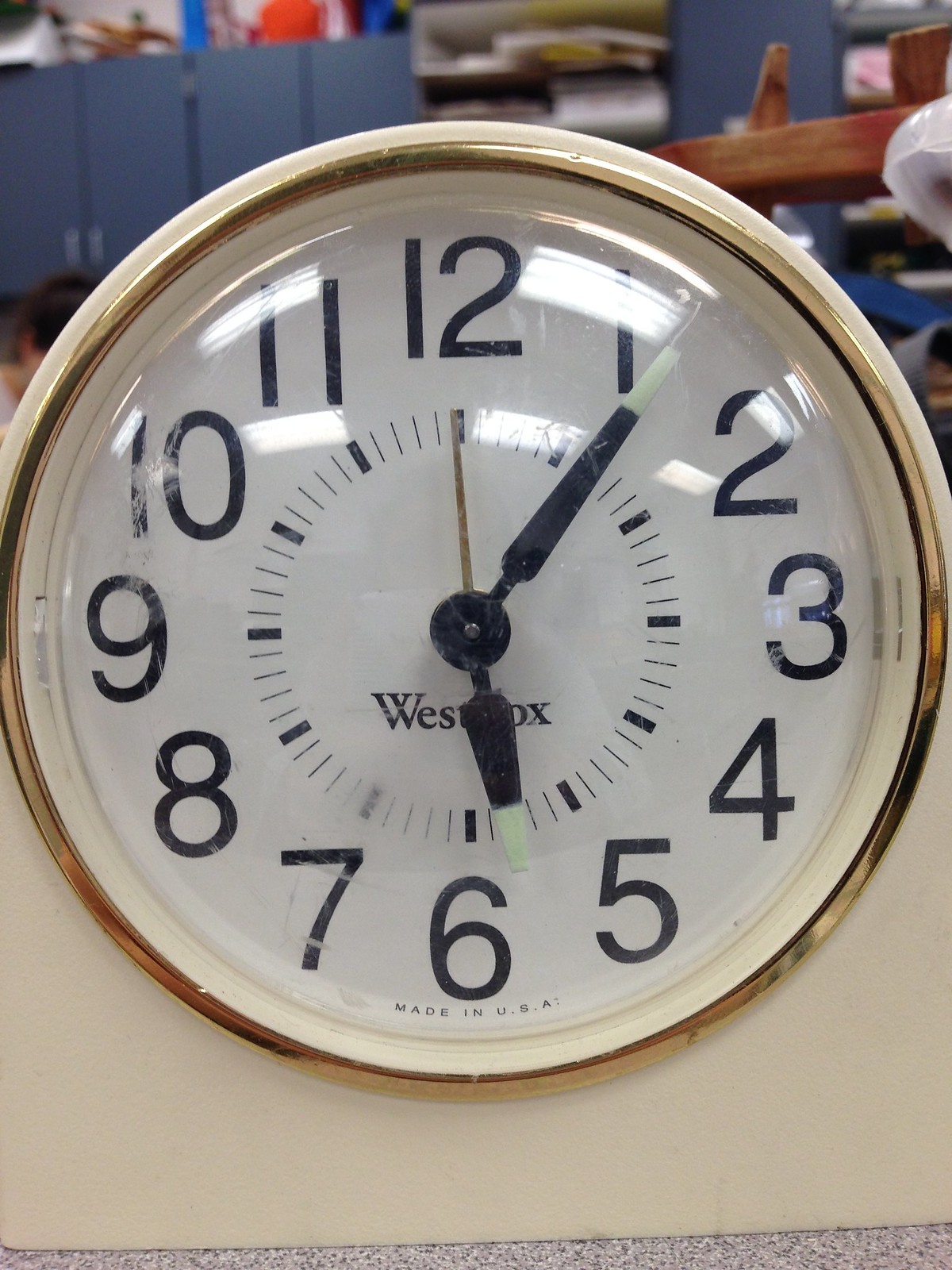This photo features a classic clock with a white face and a gold rim encircling it. Below the six o'clock position, the text "Made in the U.S.A" is prominently displayed. Beneath the clock's hands, the brand name "Westclox" is partially visible, with only "West" and "O" discernible due to the obstructing hands. At the center of the clock, the black hands transition to white near their tips, adding an elegant contrast. A slender second hand also adorns the clock, which is set to approximately 5:25. The clock is placed against a tan-colored background, with the scene further enriched by sight of gray cabinets with dual front doors and a wooden object in the backdrop.